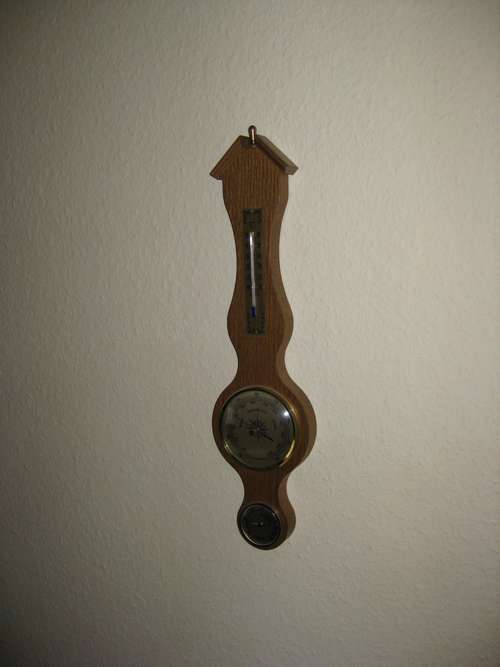A dark, atmospheric color photograph captures an antique thermometer hanging on a textured beige wall with an orange peel finish. The focal point of the image is a large wooden thermometer, characterized by its intricate design which exudes mid-century styling. The thermometer features a birdhouse-shaped top, a long neck housing the main temperature gauge, and a circular bottom that incorporates a brass-colored barometer dial with black lettering and hands, though the details are difficult to discern due to the insufficient lighting. A second circular feature is visible at the very bottom, but its purpose remains obscured in the shadows. The photograph's edges fade into blackness, further emphasizing the vintage instrument hanging there in solitude.